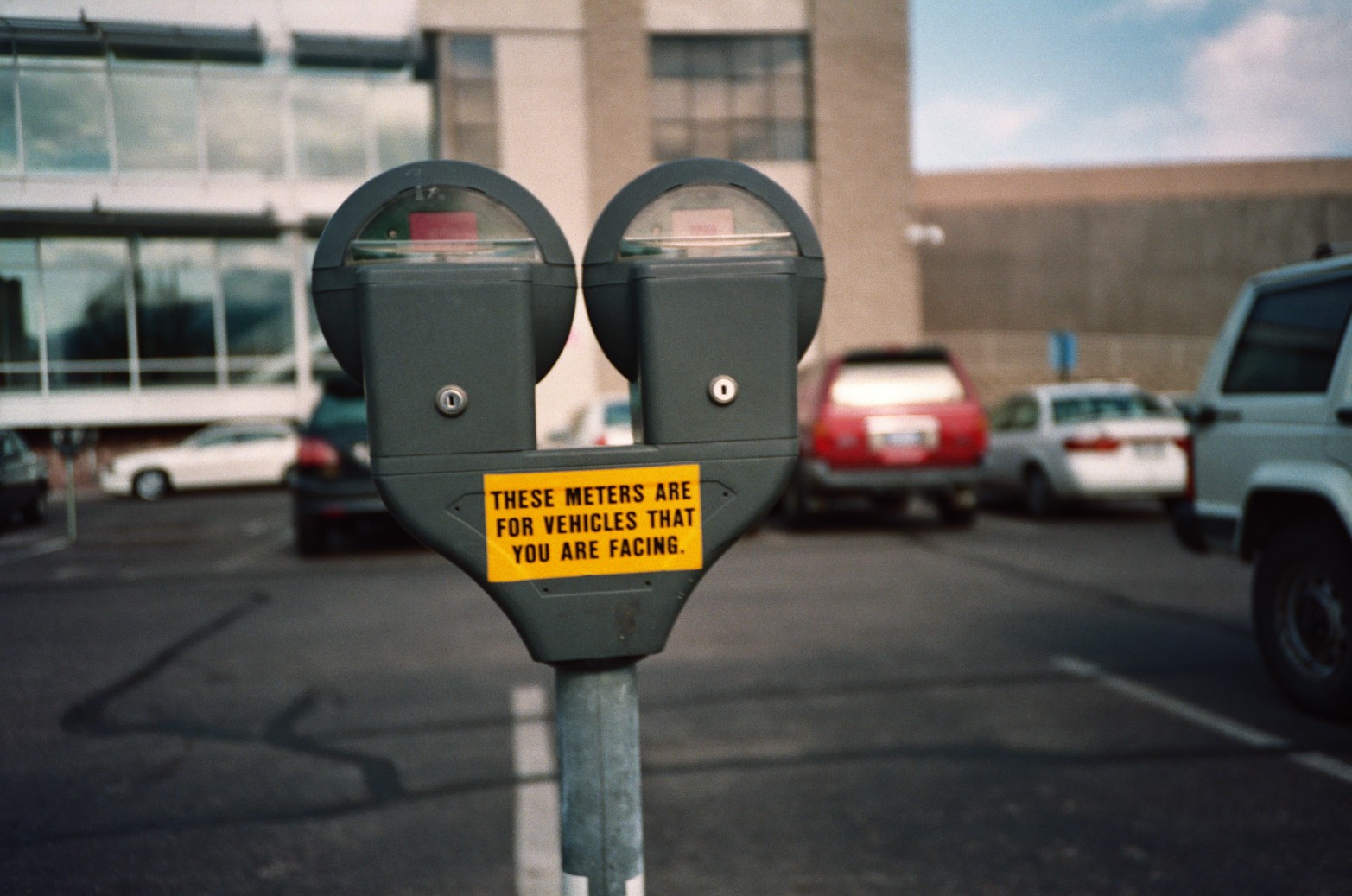This color photograph captures a daylight scene from a parking lot adjacent to what appears to be a business or office building. In the foreground, a double-headed parking meter is prominently featured, mounted on a silver metal pole. Each meter head is rounded at the top and dark grey, with a yellow sticker on the back bearing black text that reads, "These meters are for vehicles that you are facing." This indicates that drivers need to ensure they are using the correct meter corresponding to their parking orientation.

The parking lot itself is asphalt with visible white painted lines demarcating the spaces. Several cars are parked, including a white truck, a white car, a red SUV, and a dark greenish car. There's an evident organization to the parking spaces, with two spots directly in front of the meter shown as empty.

In the background, a large building with a mix of light beige brown brick and glass is visible, characterized by its numerous long windows. The presence of this building suggests it might be an office or industrial complex. Painted white accents and a glimpse of blue sky with some clouds contribute to the overall brightness and clarity of the scene.